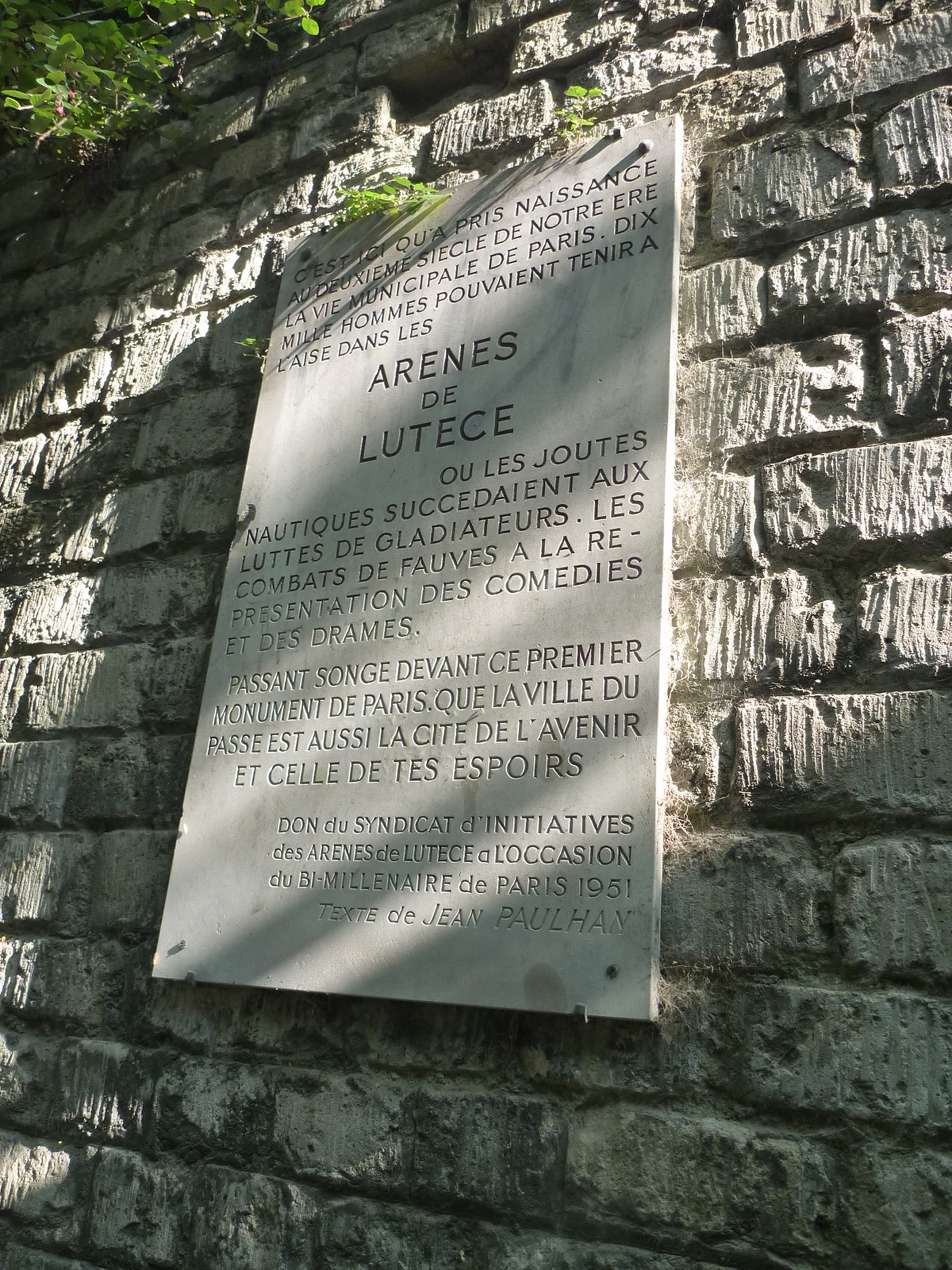The image depicts an outdoor scene featuring a rectangular stone plaque mounted on a gray brick wall. The plaque, which is etched with French text, has an enhanced structural design in its center displaying the name "Arènes de Lutèce." The surrounding environment is slightly overgrown, with vines beginning to grow on top and hanging over the edge of the wall. Cobwebs are also visible around the plaque, adding an element of neglect. The bottom of the plaque includes specific text: "Don du Syndicat d'Initiatives des Arènes de Lutèce, à l'occasion du Millénaire de Paris, 1951. Texte de Jean-Paulhan," indicating its dedication by a local syndicate in 1951 to commemorate the millenary of Paris, and attributed to a text by Jean-Paulhan. The detailed French engraving emphasizes the historical and cultural significance of the monument.